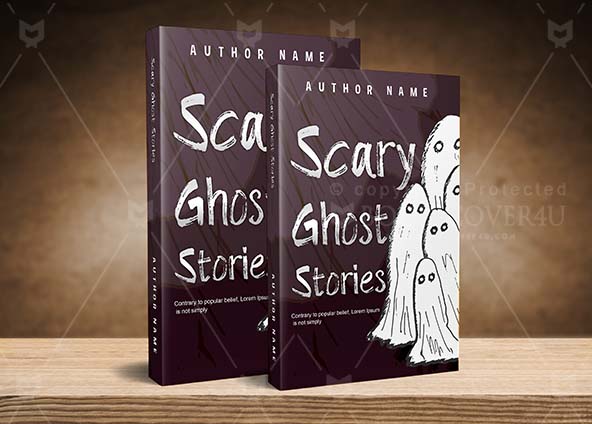The photograph showcases two identical books, titled "Scary Ghost Stories," strategically positioned on a light wooden surface with a backdrop of a dark brown, diamond-patterned wall. Both books, which feature a dark purple cover, are standing upright; the larger book is slightly behind and to the left of a smaller one. The title "Scary Ghost Stories" is displayed in a spooky white font on the left side of the covers, with "author name" written at the top. To the right, the covers depict five ghosts, resembling classic sheet-covered figures with eye cutouts, varying in height and overlapping each other. The forefront of the image includes a distinctive watermark with a crisscross diamond pattern and a cat-like symbol, further indicating it as a protected stock photo, and there are unreadable bits of text at the bottom of the cover, possibly including a website and copyright information.